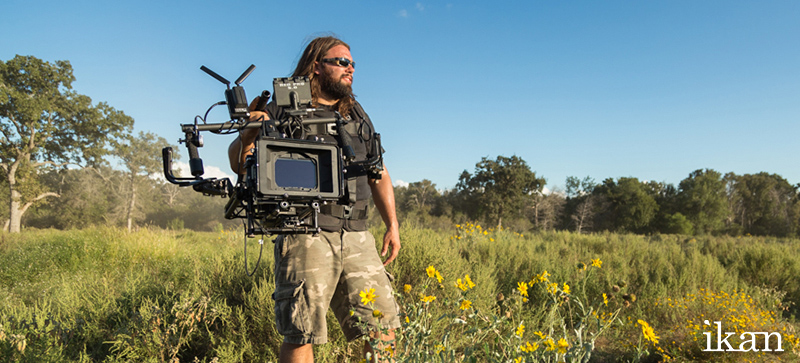A detailed horizontal rectangular image depicts a man standing in a sprawling field with knee-high to thigh-high grass interspersed with yellow flowers. He has a rugged, outdoorsy appearance, characterized by long brown hair, a thick beard, and sunglasses. His attire includes camouflage pants, a black shirt, and a vest. He appears to be in his 30s. The man is holding a large, complex piece of equipment, likely an industrial-grade movie or film camera, which features multiple screens and handles, and might be exceedingly heavy yet he holds it with one hand. The backdrop reveals a clear blue sky adorned with a mix of tall and smaller trees to the left and right, respectively. Additionally, the bottom right corner of the image displays a watermark reading "IKAN."